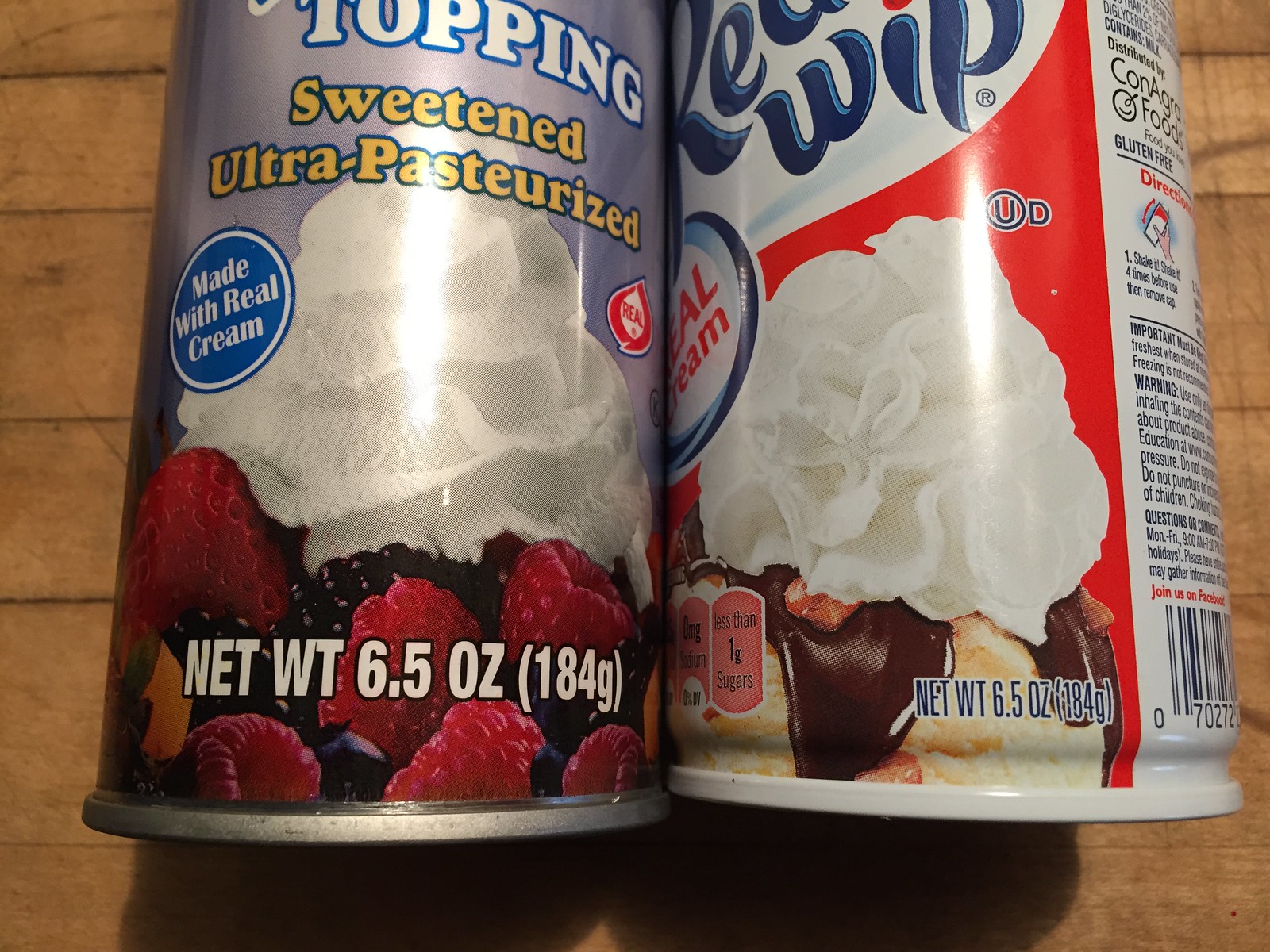This color photograph vividly captures a close-up of two food cans placed on a light wooden surface with noticeable horizontal grain lines. The composition is lit in a way that creates distinct shadows beneath the cans, enhancing the textures and depth of the image. 

The can on the left prominently features the text "Topping" in white, with "Sweetened Ultra-Pasteurized" highlighted in yellow. A circular badge on the left side states, "Made with Real Cream." The label includes an enticing image of luscious cream atop fresh strawberries. At the bottom, against a blue background, the weight is specified as "Net Weight 6.5 oz (184 grams)."

The can on the right likely belongs to another brand of whipped cream. It showcases an image of whipped cream dolloped on a donut, set against a vibrant red background. A white logo is partially visible, with the letters "K-E-W-I-P" in blue. To the left, another sign indicates "Real Cream", though only "A-L in cream" is fully visible. The far right edge of the can slightly displays the ingredients list, although the text is too small to be legible.

Overall, the photograph conveys a sense of indulgence and sweetness, with the detailed branding and appetizing images highlighting the rich, creamy contents of the cans.